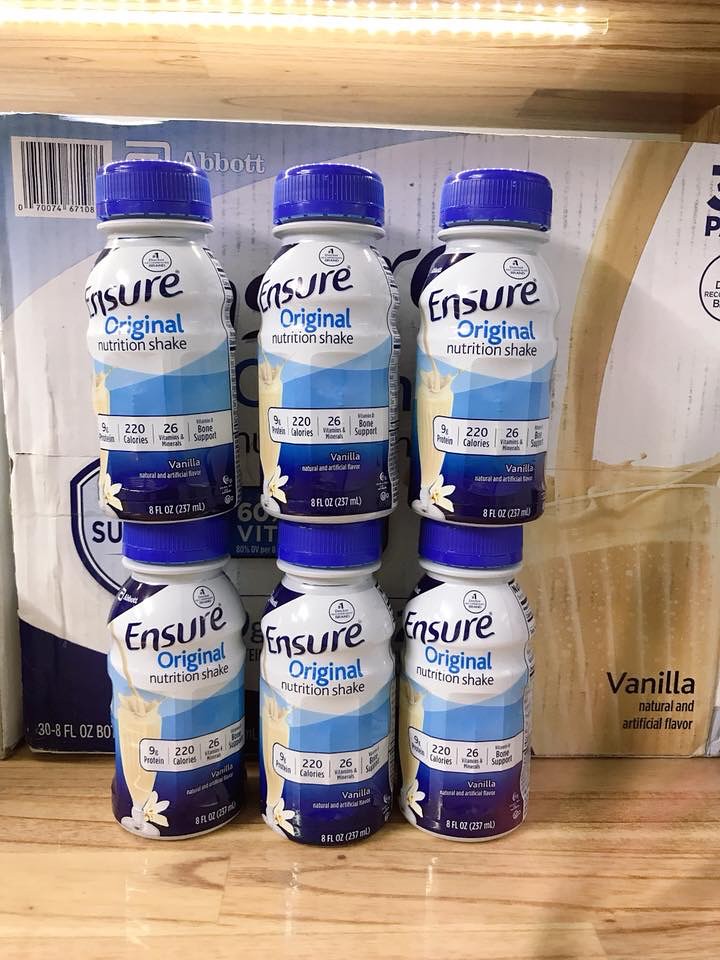This photograph features six bottles of Ensure Original Nutrition Shake, meticulously arranged in a two-tier formation. The bottom tier consists of three bottles neatly lined up side by side, while the top tier has three more bottles balanced directly above them. Behind this arrangement, a cardboard box containing the same product serves as a backdrop. The display rests on a light brown wooden surface with a distinct horizontal grain, suggesting it could be a floor or a table.

Each bottle showcases a design predominantly in white and blue, accented by a bright blue screw cap. The upper half of the label prominently displays the name "Ensure Original Nutrition Shake." Below it, the lower half illustrates a glass filled with a milkshake-like beverage, complemented by white vanilla flowers at its base, emphasizing the vanilla flavor. Additionally, nutritional benefits are highlighted on the right side of the label, outlining key information about the product's calorie content, vitamins, and minerals.